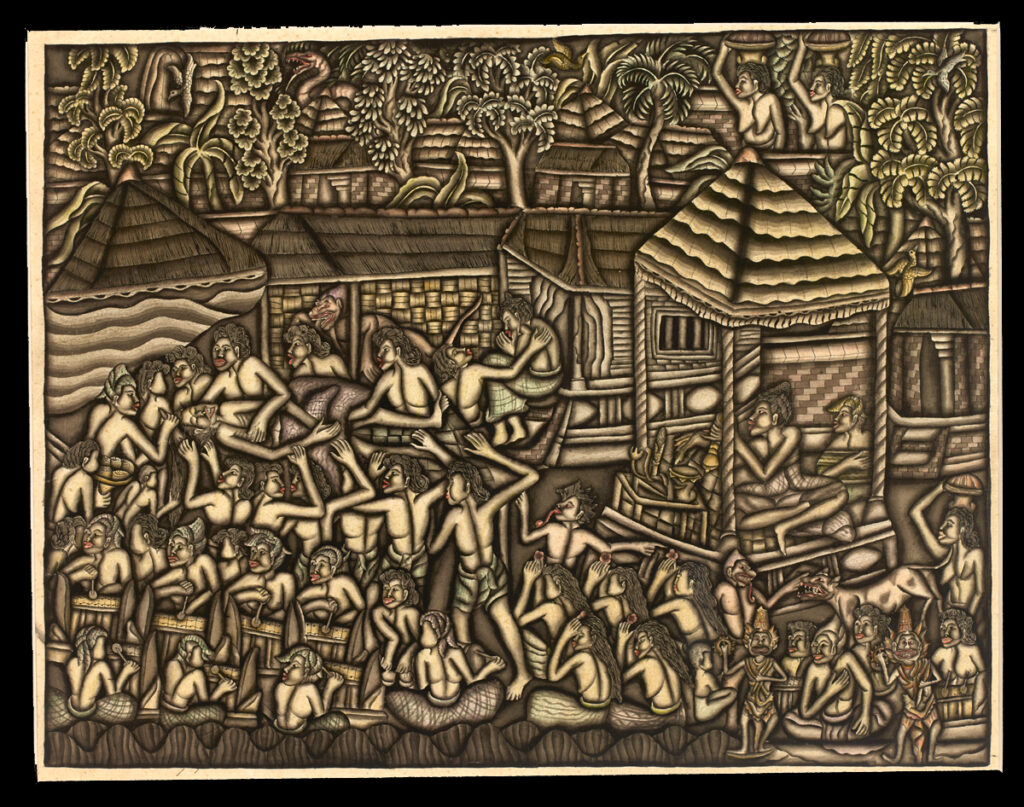The image appears to be a unique and intricate metallic pressed print reminiscent of medieval artwork, prominently featuring a village teeming with activity. The scene is characterized by island-style motifs, including huts and lush, jungle-like surroundings with palm trees and various fauna. Central to the image is a striking depiction of multiple naked individuals, both men and women. Two naked women are seen at the top, balancing baskets on their heads. Additionally, there is a group of men seemingly carrying a woman, who looks as though she is about to be sacrificed, adding an element of ritualistic poignancy to the scene. The villagers, with uniformly red lips, are drawn with meticulous detail, contributing to a monochromatic palette dominated by light brown, accented by touches of green, yellow, and potentially black, all encased in a black frame.